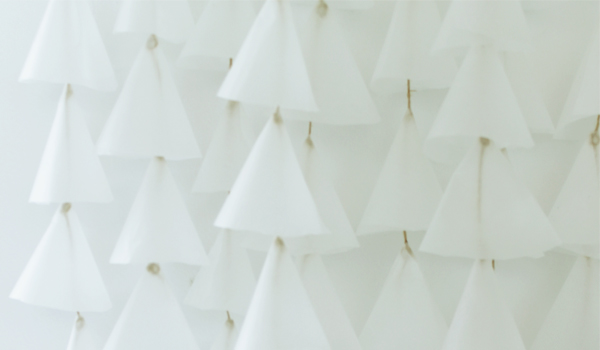The image is a color photograph featuring a close-up of what appears to be numerous strings of white, slightly translucent triangular shapes, giving an abstract and artistic impression. These triangular structures are reminiscent of delicate flower petals or abstract Christmas trees. They are arranged in roughly five vertical rows, each row featuring these white triangles stacked on top of each other. The triangles are connected by a visible brown stalk or string, which threads through their tops and occasionally peeks through between them. The backdrop of the image is entirely white, creating a minimalist and dreamy aesthetic. There are no discernible people, animals, writing, or mechanical objects within the frame, emphasizing the simple yet intricate details of the hanging triangular forms.